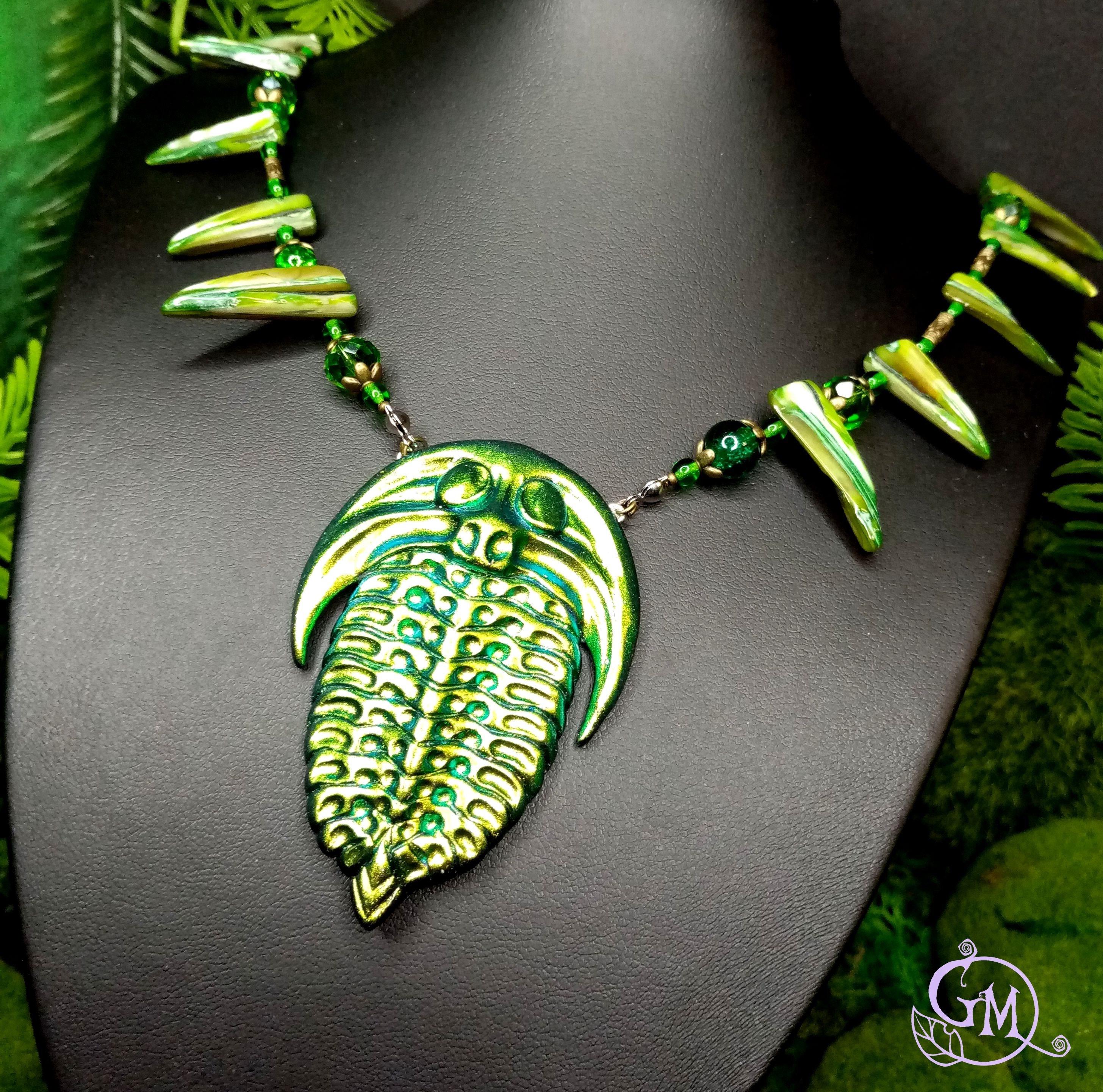Amidst a lush green backdrop of vibrant leaves, this advertisement prominently features a striking necklace displayed on a black mannequin headpiece. The necklace, adorned with shades of green and gold, features a central charm that appears to be an intricate piece resembling a mix between a pineapple and a peanut, complete with eyes and a small nose crowned by an upside-down crescent moon. Surrounding this main charm are bead-like elements that evoke the appearance of fangs or alligator teeth. In the bottom right corner of the image, the GM logo in lavender serves as a subtle yet noticeable brand mark.